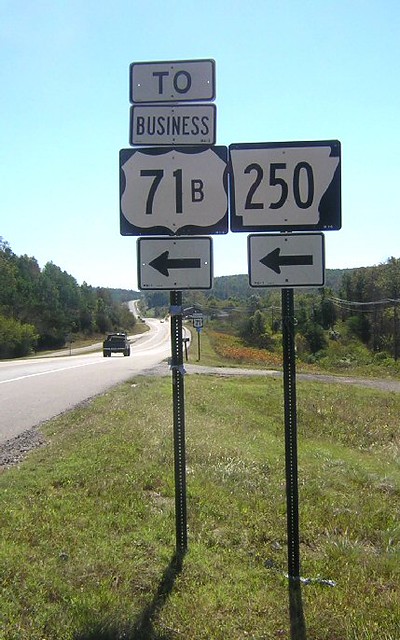This daytime photograph captures a stretch of highway bordered by lush, thick green trees on both sides, with a clear blue, mostly cloudless sky overhead. In the foreground, situated on green grass, are two metal poles with several road signs mounted on them. The closest pole, a little to the left of center, supports a rectangular white sign outlined in black with "2 TO" written in capital letters. Directly below it, another rectangular white sign, similarly outlined, reads "BUSINESS" in black. Further down, a square sign features a black badge symbol with "71B" in bold letters. Adjacent to these, the second pole holds a square sign with a black outline depicting a state shape and the number "250" inside it, along with a directional arrow pointing left. Another square sign below this also bears a black directional arrow pointing left. You can observe a dark-colored truck driving away on the highway, which is marked with a white line. The background reveals more trees lining the horizon.